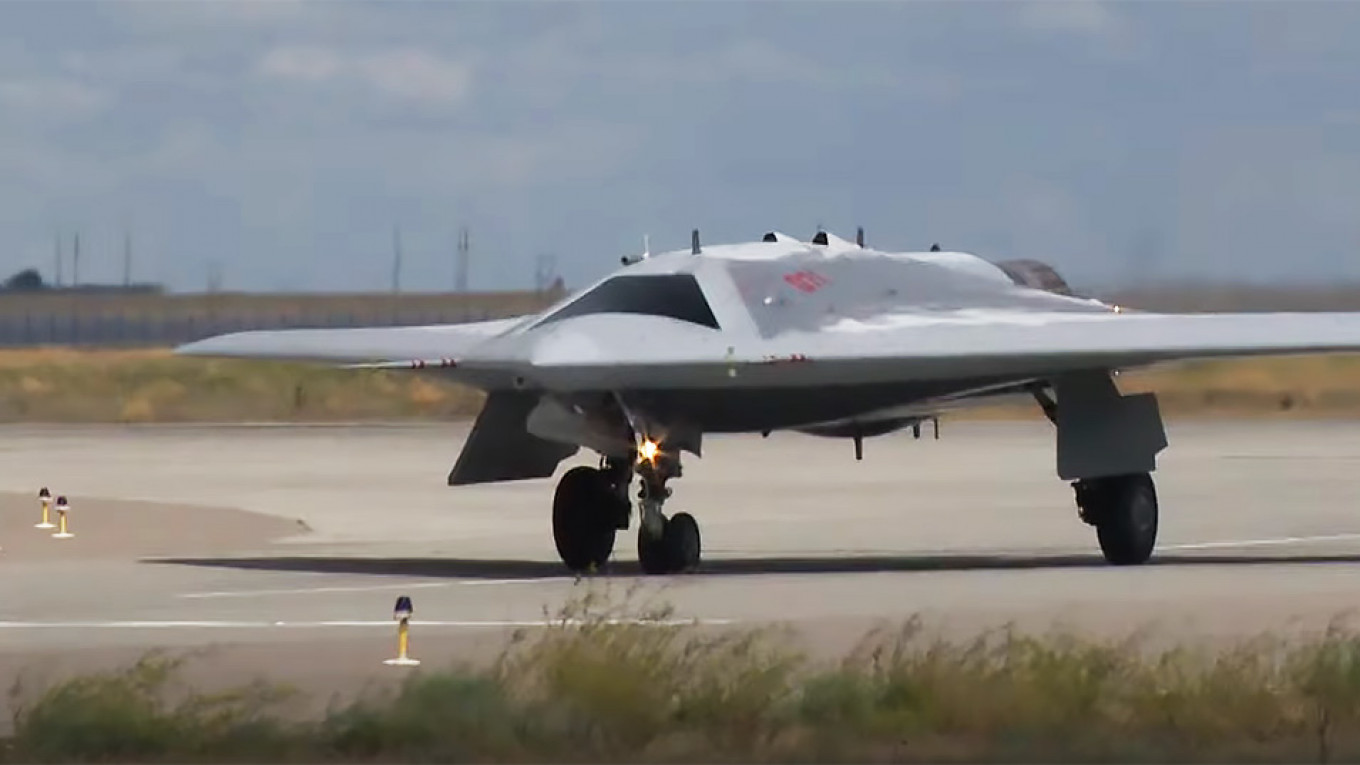The photograph captures a sleek, gray, military-style stealth plane with a low, flat design and a black windshield. It is taxiing on a runway, evident from its extended landing gear and a slight forward roll. The plane, predominantly gray with some small red markings and a bottom light, stands out against the natural daylight. The background reveals a blurred blue sky with scattered clouds, power lines, and a hangar-like building visible in the distance. The runway scene is enhanced by the surrounding dry grass and pavement lights, emphasizing the aircraft's poised readiness for takeoff or its completion of a landing, situated within a depicted military base.